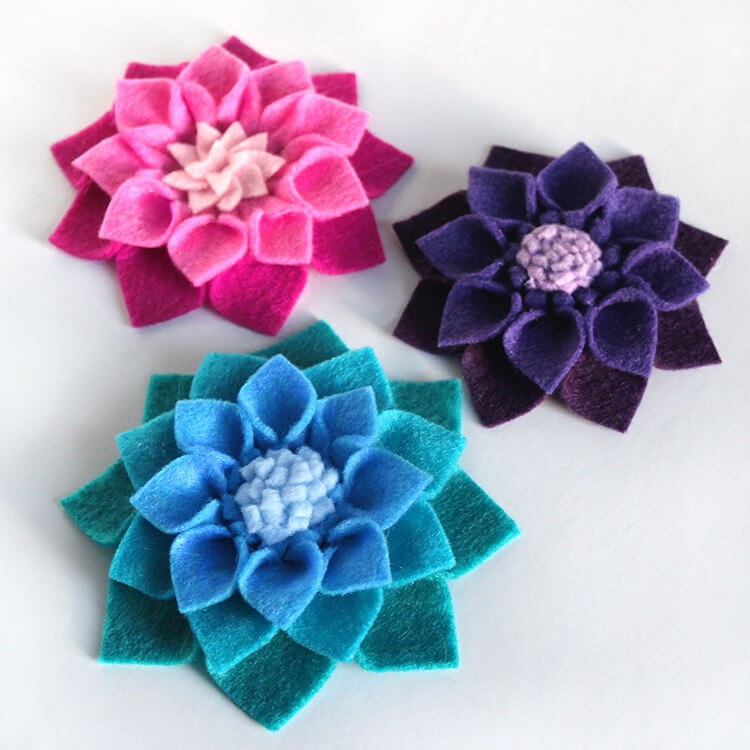In this image, three intricately handmade felt flowers are displayed on a light gray background. Each flower showcases a distinct color palette and construction, offering a vivid spectrum of artistic detail. 

The first flower, positioned to the top left, combines hues of pink and a deeper rose, featuring an off-white center composed of tiny petal-like structures. The middle flower presents a striking contrast with its dark blue gradually transitioning to a lighter blue, and its center adorned with small beads. The third flower, a study in turquoise and pale blue, is distinguished by its centrally clumped smaller petals, resembling the structure of a dahlia. 

All three flowers appear to be meticulously crafted from felt, either glued or sewn together, and may function as decorative pins or corsages, enhancing the elegance of a sweater or outfit. Each flower's center is distinct, adding to the overall charm and suggesting a thoughtful, handmade touch that results in a visually captivating arrangement.